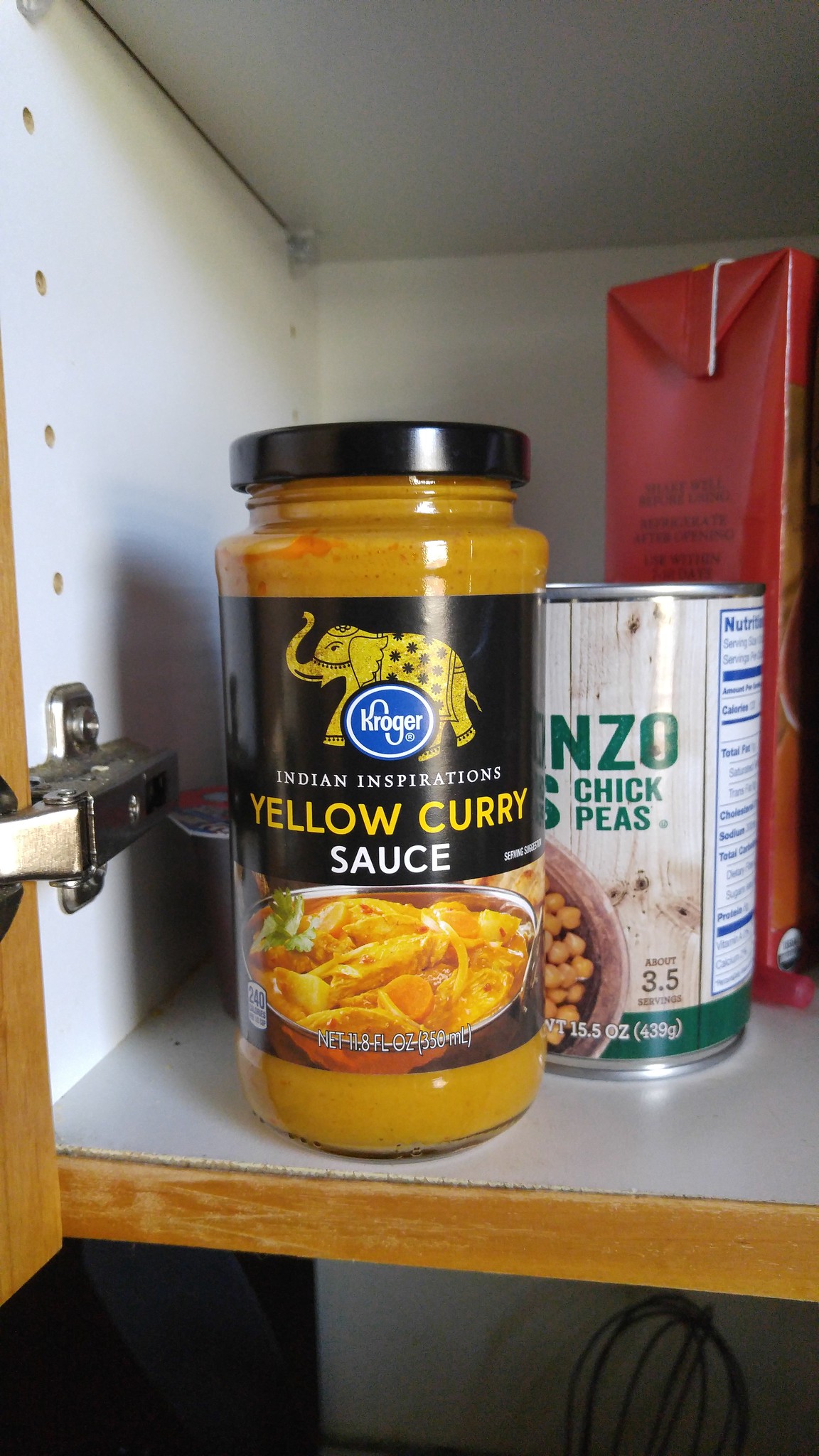This photograph captures the interior of a kitchen pantry cabinet door, which is part of a small, light brown wooden cabinet equipped with a metal bar mechanism for opening and closing. The inside of the cabinet is painted white, providing a neat contrast to the light brown exterior.

On what is likely the counter surface beneath the cabinet, a whisk is visible. Within the pantry space, a jar of yellow curry sauce takes center stage. The label on the jar features the term "Yellow Curry" in prominent yellow letters, "Sauce" in white letters below it, and the phrase "Indian Inspirations" also in white letters above. The Kroger grocery store emblem is displayed — a blue background with a white circle framing the name "Kroger" in white letters. Further adorning the label is an illustration of a yellow elephant decorated in traditional Indian attire.

The sauce inside the jar appears to be medium yellow and creamy, matching the food shown in a pan illustration at the bottom of the black label. The jar itself is topped with a black lid. Positioned behind the jar is a can of chickpeas marked "3.5," and beyond that, a cardboard-type container designed to hold liquid.